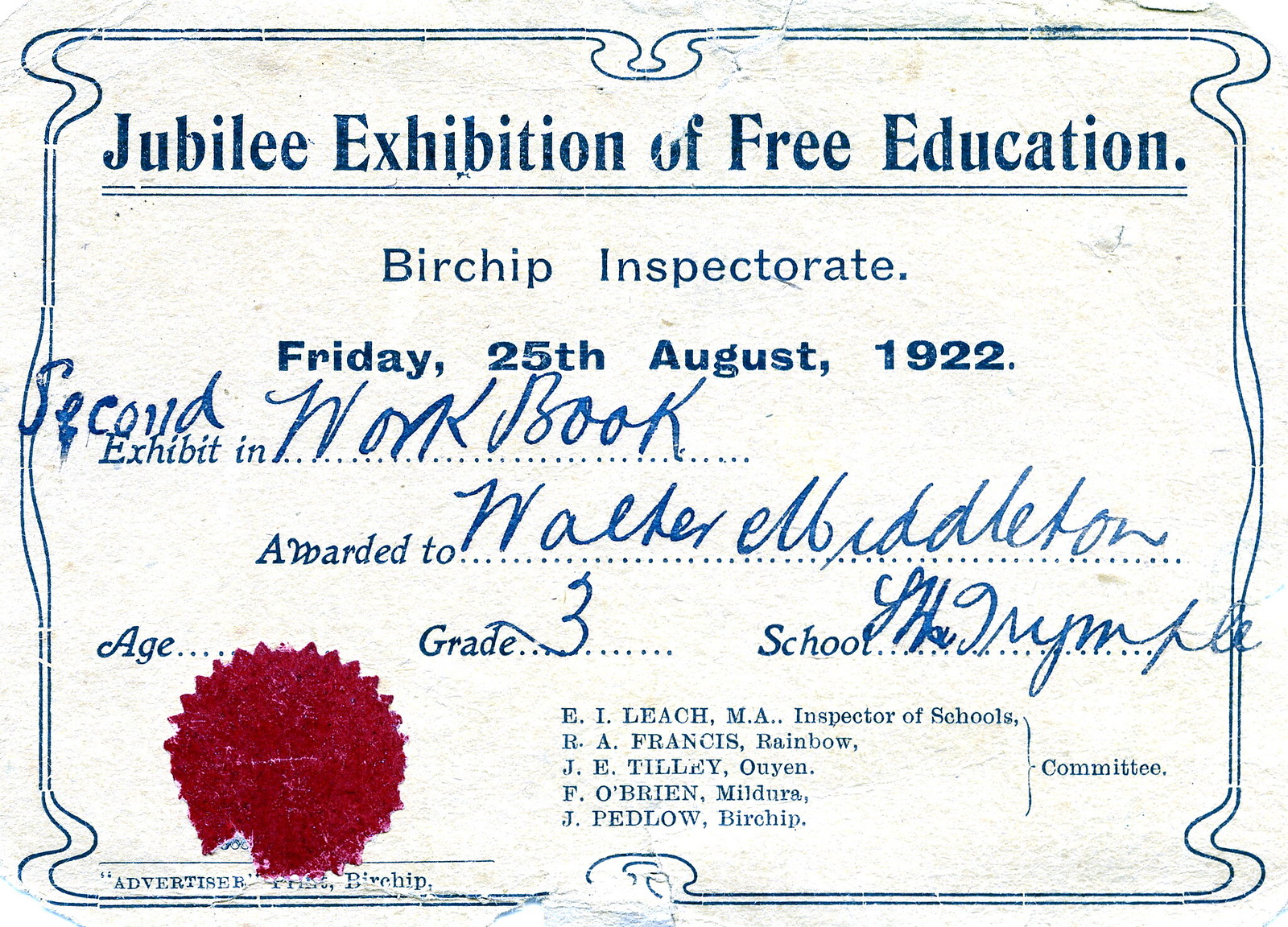The image is of a vintage certificate on old, off-white paper with a decorative blue, squiggly frame around it. At the top, the text is in blue font and reads "Jubilee Exhibition of Free Education" with two horizontal lines underneath. Below that, it mentions "Birchip Inspectorate" and the date "Friday, 25th August, 1922." The certificate is awarded to "Walker Matterton" for an exhibit in a second workbook. The age section is blank, and he is listed in grade three. The school's name is written in an undecipherable cursive. Beneath this, the certificate lists the committee members, and there is a red stamp in the bottom left corner. The overall design shows signs of aging and the paper appears tattered.